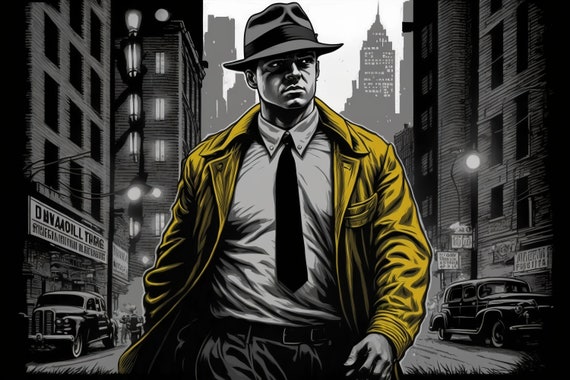In this striking, noir-inspired comic book illustration, a man resembling an FBI agent or 1940s private detective walks down a city street at night. He dons a gray and black fedora, a yellow trench coat, a black tie, and gray pants, casting a stoic yet vigilant gaze to his left. The background reveals an urban landscape with several buildings, including a several-story-high gray structure with an unclear sign that seems to read "DMV" and an indistinct tire advertisement. The bygone era is further accentuated by classic 1930s and 1940s cars parked on both sides of the street. The dark surroundings are punctuated by streetlights, one of which illuminates a rundown building on the right. Skyscrapers, including one that looks like the Empire State Building or possibly the Chrysler Building, rise in the distant background, standing against a stark white sky. This vivid scene feels almost lifelike, capturing the essence of a vintage detective story with meticulous detail.